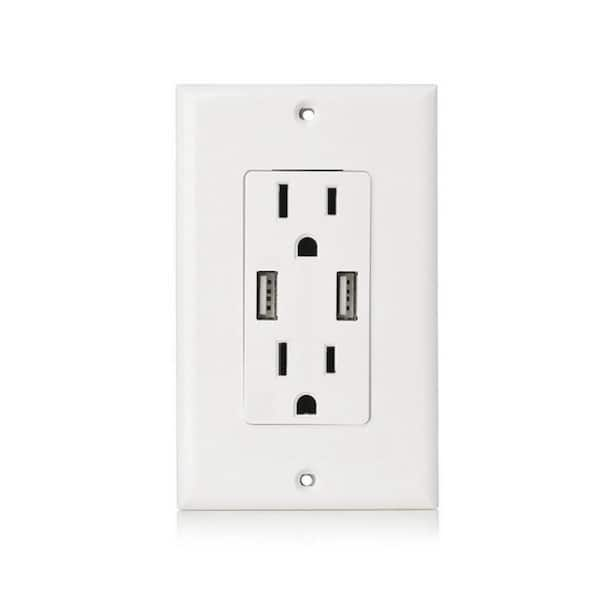The image depicts a white electrical outlet commonly found in homes or buildings, designed for both three-prong plugs. The outlet plate features two vertically oriented receptacles, each with two straight slots above a semi-circular grounding hole. The receptacles are positioned with one at the top and one at the bottom, mirroring each other. The central panel, which is gray, contains four small, pinhole-like square slots, possibly for additional connectivity options, such as charging devices directly via USB. Surrounding the outlets is a rectangular frame with two screw holes—one at the top and one at the bottom—for securing the plate to the wall. This kind of outlet plate may also include ground fault circuit interrupter (GFCI) protection, enhancing electrical safety. The image background is white, suggesting it might be styled for a sale listing, possibly on a platform like Home Depot or Lowe's.